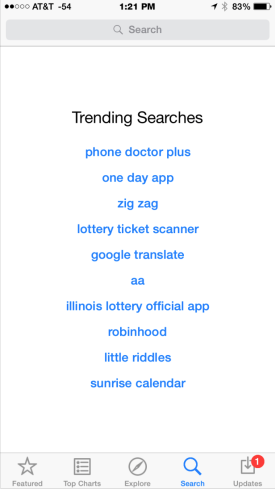This image displays a screenshot of a mobile phone or tablet app showcasing trending searches. At the top left, there's a signal strength icon rated at two out of five dots, likely indicating a weak network connection, accompanied by the label "AT&T" and a signal strength of "-54." At the center of the status bar, the current time is displayed in bold black font as "1:21 PM." On the top right, there is a diagonal right arrow, a Bluetooth symbol, a battery level of "83%" with its icon, suggesting connectivity and battery status.

Below the status bar is a gray search bar featuring a magnifying glass icon and the word "Search." The section below is titled "Trending Searches" in black text, listing popular search terms in blue font: "Phone Doctor Plus," "One Day App," "Zigzag," "Lottery Ticket Scanner," "Google Translate," "AA," "Illinois Lottery Official App," "Robin Hood," "Little Riddles," and "Sunrise Calendar."

At the bottom of the screen, a navigational gray bar provides options including "Featured," "Top Charts," "Explore," "Search" (currently highlighted in blue), and "Updates." Notably, "Updates" has a red circle with the number "1," indicating one pending update.